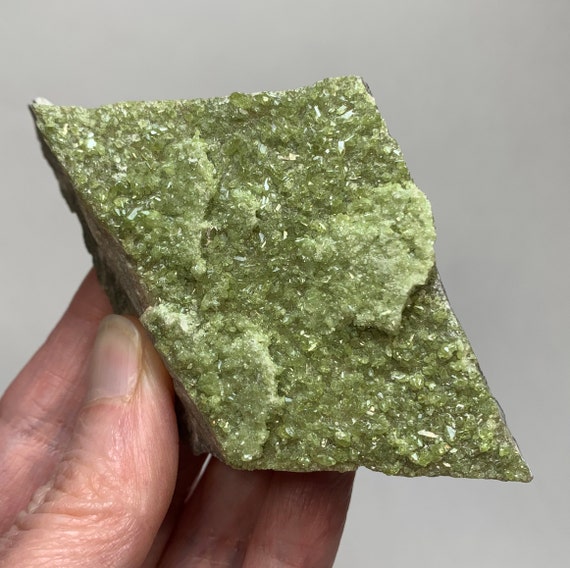In this image, we observe a Caucasian hand, likely belonging to an older individual over the age of 40, holding up a greenish mineral. The background is a simple, light plain gray, making the foreground details more prominent. The hand has a light complexion with a slight reddish hue and visible wrinkles. Notably, the fingernails are fairly long and somewhat dirty. The fingers, including the thumb, index, middle, ring, and pinky, are bracing and supporting the mineral mainly from the left side of the image. 

The mineral itself is not emerald but another green mineral. It has been cut into a rectangular shape, closely resembling a parallelogram, with relatively flat surfaces that are slightly uneven. The surface facing the camera is adorned with small sparkling light green crystals and features noticeable lumps containing these crystals. The rest of the stone appears to be a grayish color. The texture of the mineral's surface is highlighted by the light or flash used in the photograph, giving it a rough appearance.